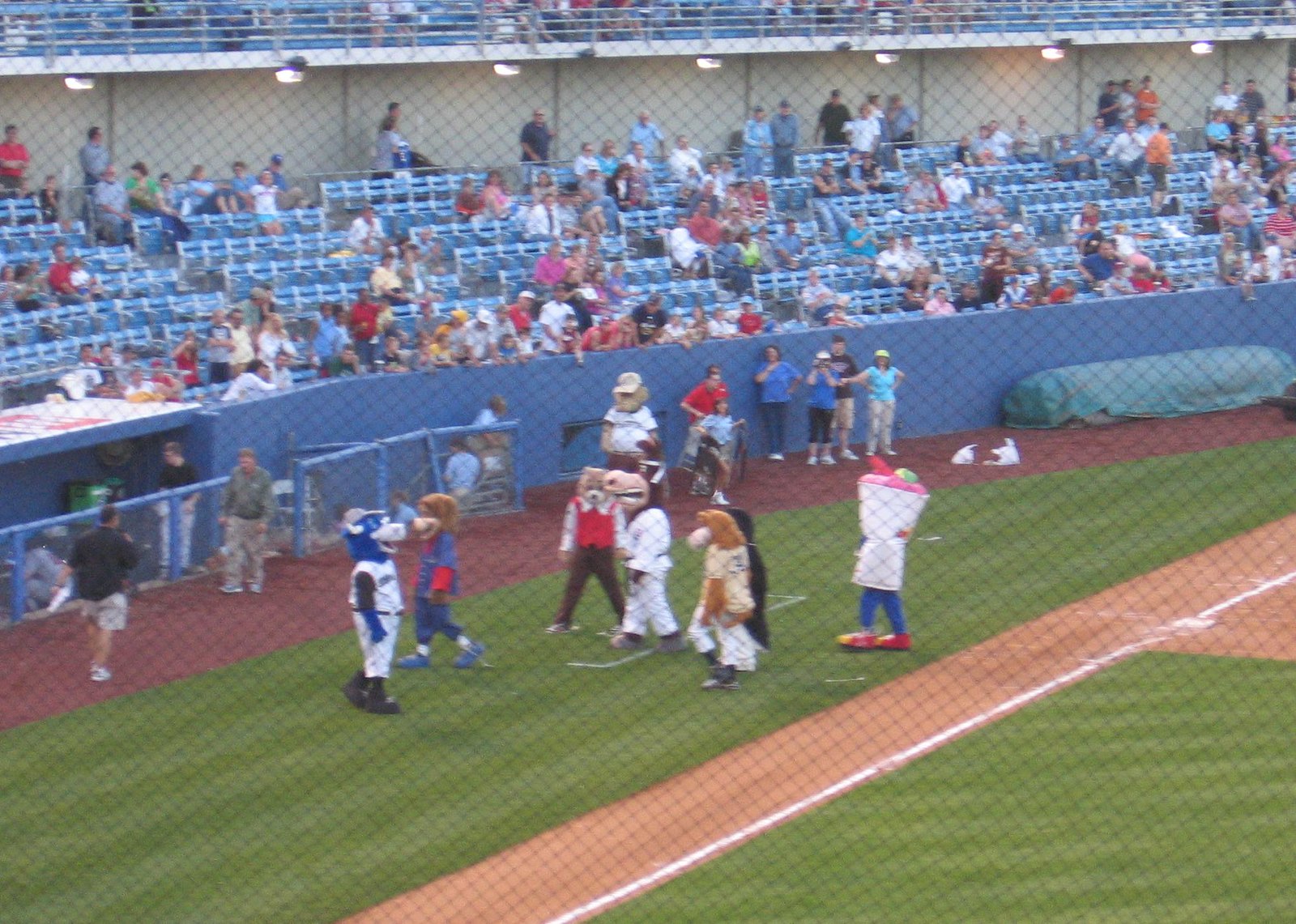The image is a detailed photograph of a baseball field, captured through a chain-link fence, featuring the classic tan-brown clay sand typical of such fields. The meticulously manicured, uniform-height grass on either side frames the shot, leading to the central focus: a gathering of multiple mascots around the circumference of the baseball pitch, near the dugout area.

These mascots, designed in anthropomorphized styles, include a blue bull, a dog in a karate suit, and a blue pants-wearing, red-shoe-clad cup mascot that appears to be holding a pink slushy or ice cream. Additionally, a lion in a white baseball suit adds to the vibrant assembly. Behind them, portions of the seating stands are visible, showing rows of blue chairs against an off-white wall with lights on each partition. The crowd, scattered sparsely, suggests an American city with a modest attendance, though a fraction of the bottom level seats are occupied.

A blue short fence leads toward the dugout where a dark brown patch area with a tarp under a green cover can be seen to the right. This overall composition paints a vivid and lively scene of a baseball stadium, absent of players, but bustling with mascot activity and engaged spectators.